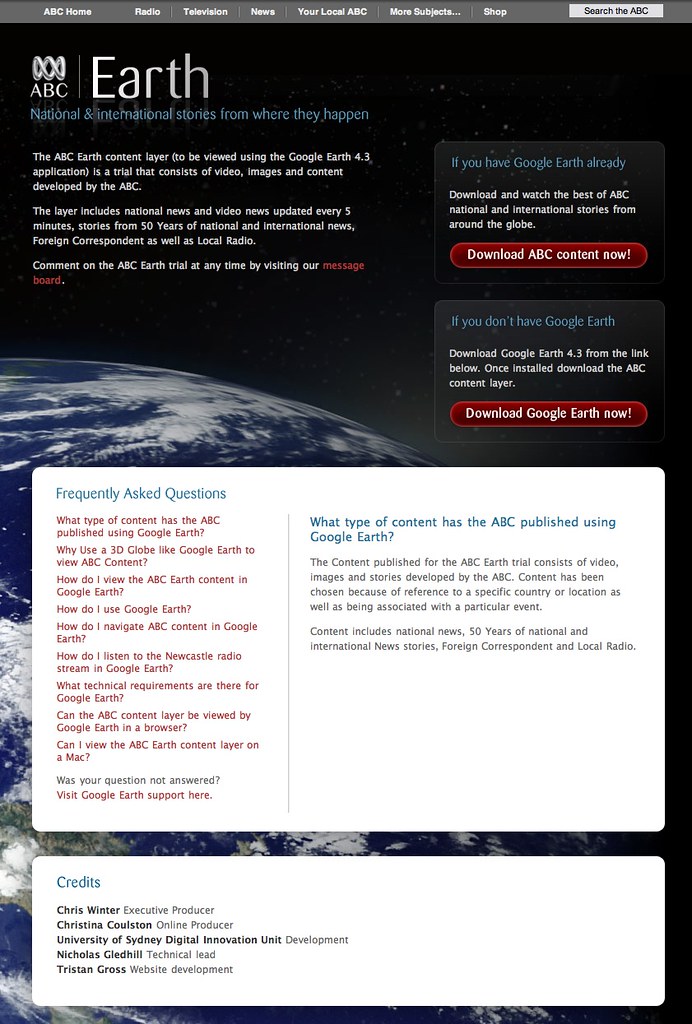This is a caption that somebody gave for an image using their voice. Clean it up and formulate it into a descriptive caption. Make it very detailed.

This is a website and the top strip is gray and on the left it says ABC home Then it says radio television news your local ABC more subjects dot dot dot shop And then on the right search ABC in a data field that is white That's all right writing on a gray background then below it says on the black background ABC Earth National and international stories from where they happen and below that it says the ABC Earth content layer to be reviewed using Google Earth 4.3 Application is a trial that consists of videos images and contacts developed by ABC The layer includes national news video news update. It's every five minutes stories from 50 years to national and international news Foreign correspondence and as well as local radio comment on the ABC Earth trial at any time by visiting our message board That's red On the right of that it says if you have Google Earth already Download and watch the best of ABC national international stories for around the globe and there's a red button that says download ABC content now Below that it says if you don't have Google Earth download Google Earth 4.3 from the link below once installed out installed download the ABC content layer Download Google Earth now is in white on a red button Below that there it says frequently asked questions

---

At the top of the website, a gray navigation bar features the ABC logo on the left, followed by links labeled "Home," "Radio," "Television," "News," "Your Local ABC," "More Subjects…," and "Shop." On the right side of the bar, there is a white search field with the label "Search ABC."

Beneath the navigation bar, against a black background, a banner reads: "ABC Earth - National and International Stories from Where They Happen." Below this banner, a description explains that the ABC Earth content layer is being reviewed using Google Earth 4.3. This trial application includes a collection of videos, images, and articles developed by ABC. The content includes national news, video news updates every five minutes, stories from the past 50 years, national and international news, foreign correspondence, and local radio segments. Users are encouraged to comment on the ABC Earth trial by visiting the message board, which is highlighted in red.

To the right, a section prompts users who already have Google Earth to download and watch ABC's best national and international stories. A prominent red button reads "Download ABC Content Now."

Below this, there is information for users who do not have Google Earth. It instructs them to download Google Earth 4.3 from the provided link and then install the ABC content layer. Another red button reads "Download Google Earth Now," with the text in white.

At the bottom of the section, there is a link labeled "Frequently Asked Questions."